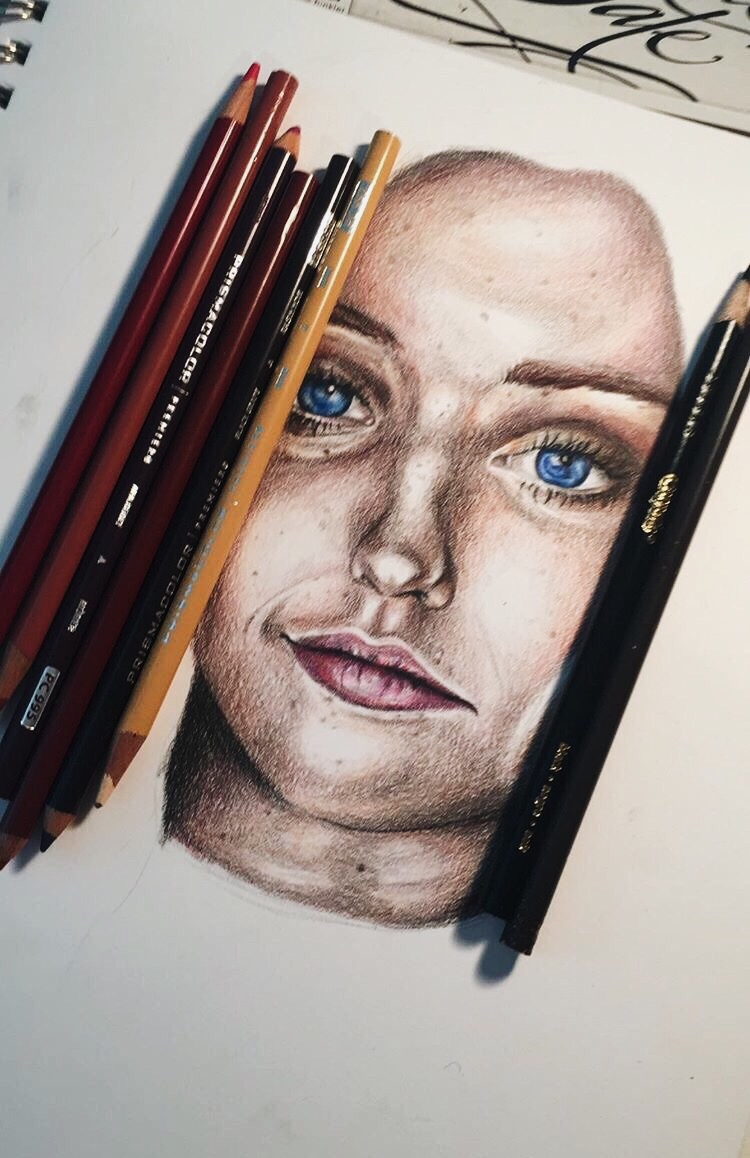The image is a detailed sketch of a realistic human face and part of the neck, drawn diagonally on white paper. The neck extends towards the bottom left-hand corner, while the head tilts to the right. In the upper right-hand corner of the paper, the word "A-T-E" is written in an elegant script. The paper itself is from a spiral notebook, with visible square holes along the upper left-hand edge through which silver spirals thread.

The sketch is surrounded by colored pencils. On the right side of the face, two pencils, appearing to be shades of black, are visible. On the left side, six colored pencils in varying shades of reds, browns, and a yellow are scattered. The subject's gender is ambiguous, but there are features suggesting it might be a female. The person has fair skin, blue eyes, brown eyebrows, and a pointy nose. The lips have a subtle pink hue, possibly indicating lipstick. Additionally, there are distinctive beauty marks on the neck, with three marks clearly visible.